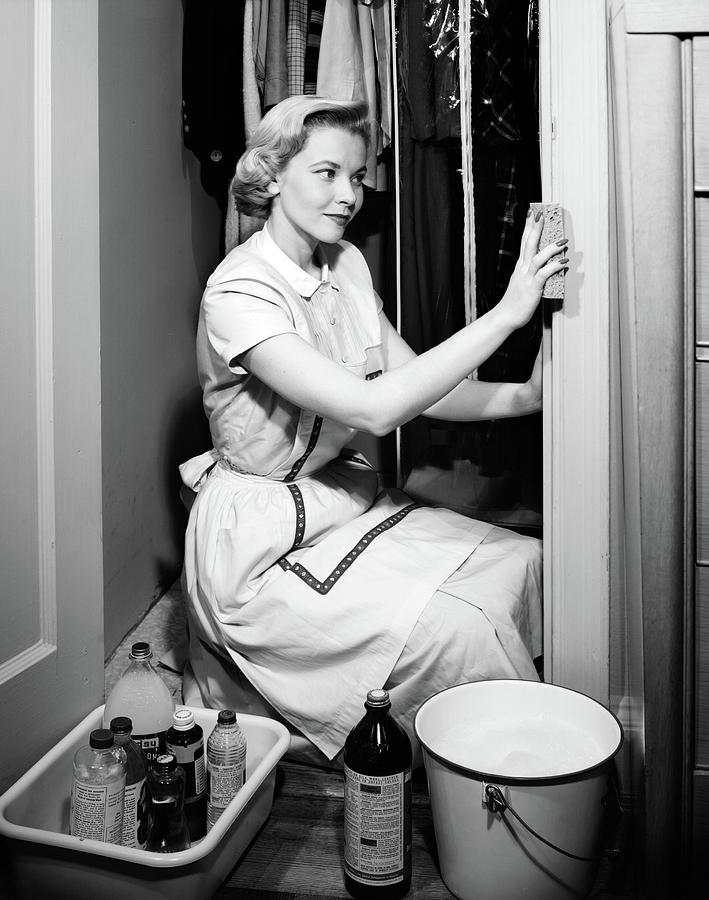The black-and-white photograph captures a staged indoor scene, evocative of the 1950s. It features a Caucasian woman with short, wavy blonde hair, styled in a typical 1950s fashion. She is dressed in a long dress with short sleeves and a white collar, over which she wears a white apron. She is kneeling inside a closet, evident by the long draped clothes hanging behind her, some protected in plastic wrap.

She is engaged in cleaning, using a sponge to scrub the frame or wall of the closet on her right. Her painted fingernails are visible as she works. In front of her, near her right knee, sits a large white metal bucket. Next to the bucket, there is a black bottle, and beside it, a white plastic tub containing several glass bottles, all with their caps on. The closet door on the left, noticeable by its indents, adds to the domestic feel of the image. The careful composition and artificial lighting highlight the meticulous details, reinforcing the staged nature of the photo.